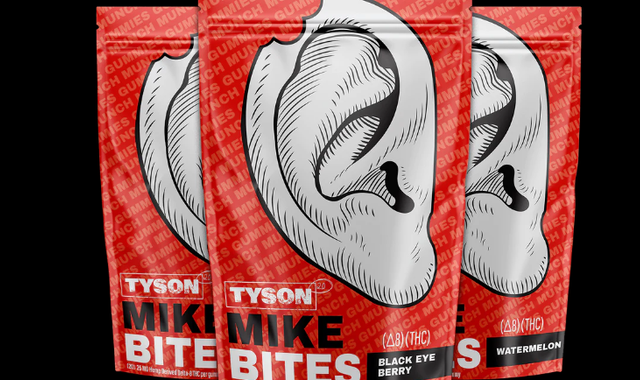This image depicts three red, resealable packages of THC edibles called "Tyson Mike Bites," a playful nod to famous boxer Mike Tyson. The front of each bag features a large, cartoonish graphic of an ear with a bite taken out, referencing Tyson's infamous fight with Evander Holyfield. Each package prominently displays the product name "Tyson Mike Bites" and includes the term "THC," confirming the presence of the psychoactive compound. The background of the packaging is decorated with slanted, transparent text that reads "gummies" and "munch." Flavors noted include "Black Eye Berry" and "Watermelon," although the third flavor remains obscured. The overall background of the image is black, making the red packages stand out distinctly. These Delta-8 THC gummies are arranged with one bag in the center and two partially hidden behind it, emphasizing the ear graphic and playful branding.